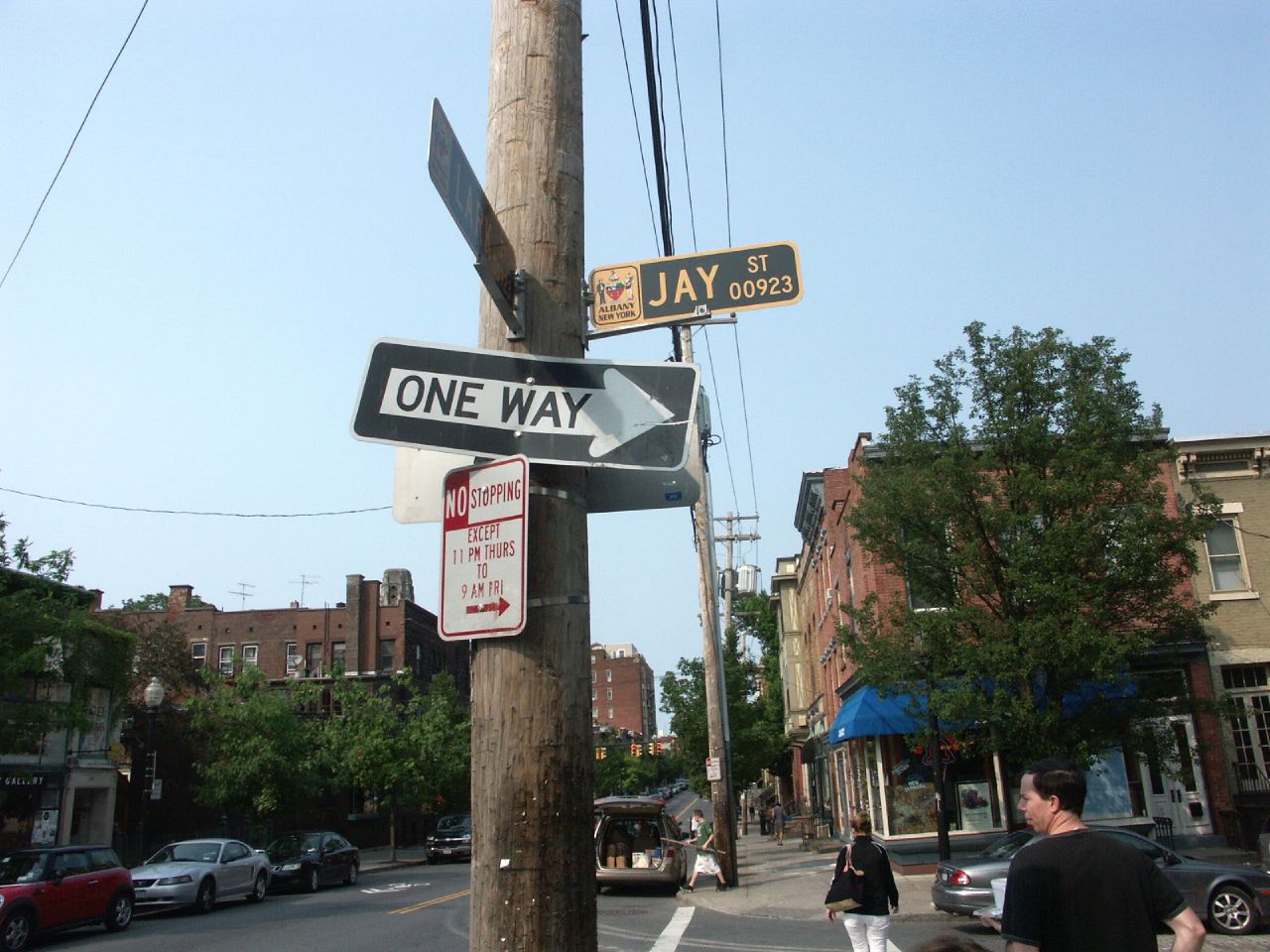The image captures a bustling suburban street scene in Albany, New York, featuring several distinct elements. Dominating the scene is a wooden telephone pole equipped with various signs: a prominent street sign indicating J Street, 00923 with yellow text on a black background, a white one-way sign pointing to the right, and another sign prohibiting stopping except from 11 p.m. Thursday to 9 a.m. Friday. Adjacent to the street sign, there is a sticker indicating Albany, New York, possibly containing a local symbol.

The background features a clear blue sky enhancing the visual appeal. The environment is a mix of residential and commercial buildings, many constructed from brick, with one exhibiting a blue awning. Vehicles are parked along the street including a noticeable red Mini Cooper. On the left side of the image is a lamppost with a white bulb.

At the bottom right, two people are seen crossing the crosswalk; one individual holds a stick and is either putting items in a van or adjusting their white skirt, while another person crosses behind them. A tree adorns the sidewalk, adding a touch of greenery to the urban setting.